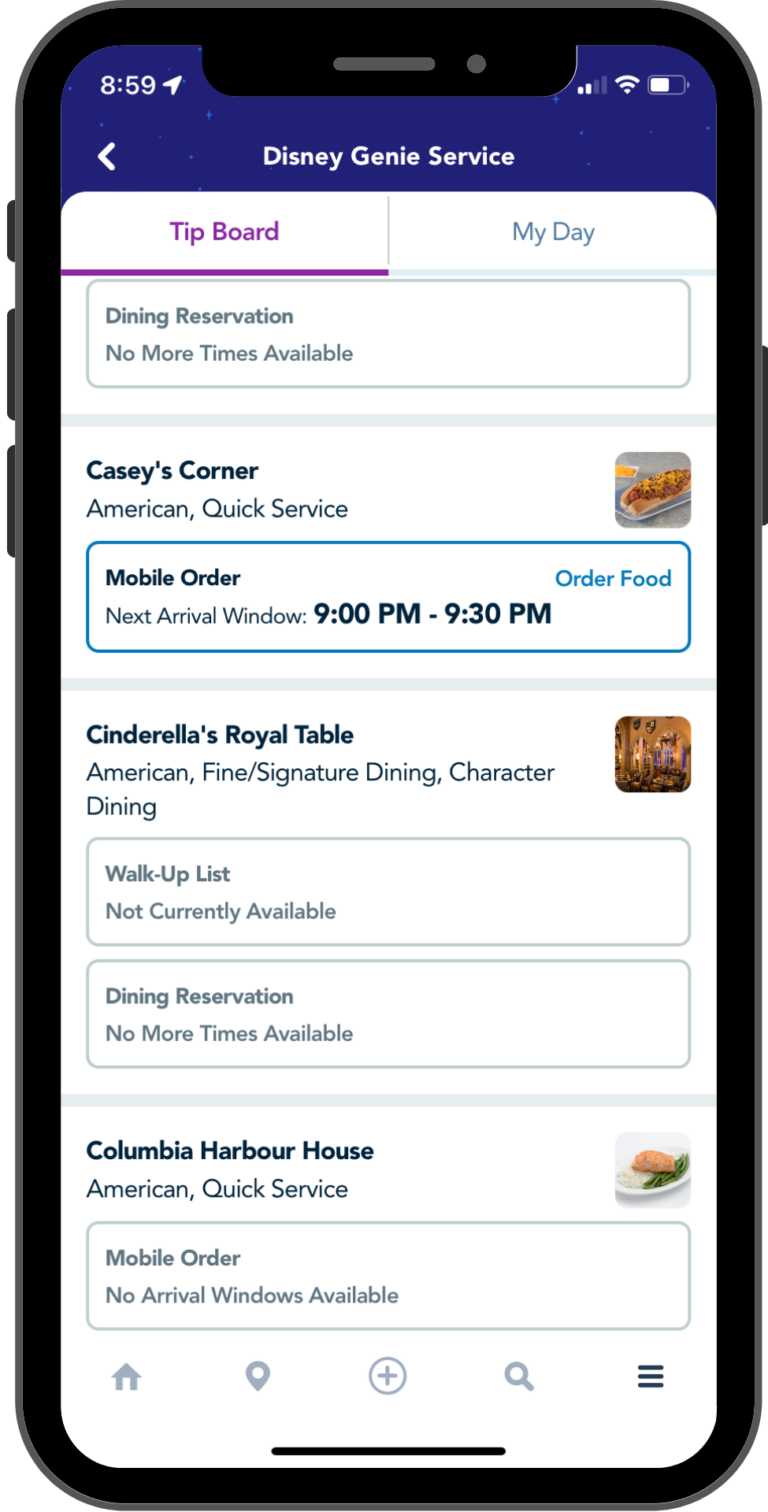The image showcases a black cell phone positioned against a solid white background. On the left side of the cell phone, three buttons are visible, while the right side features a single button. The phone's screen is active, displaying an interface presumably related to the Disney Genie service. 

At the top right corner of the screen, set against a blue background, the signal strength shows two out of four bars, the Wi-Fi icon is illuminated, and the battery indicator appears three-quarters full. The time displayed in the top left corner reads 8:59.

Beneath the status bar, the interface features two white boxes labeled "Tip Board" on the left and "My Day" on the right. Below this section, there's an announcement for "Dining Reservation" stating that no more times are available. 

Further down, the screen showcases bold text for "Casey's Corner," an American quick-service restaurant, indicating that the next mobile order arrival window is from 9:00 PM to 9:30 PM with an option to "Order Food."

Lastly, the screen mentions "Cinderella's Royal Table," an American fine signature dining experience with character dining. It states that the walk-up list is not currently available and that there are no more times available for dining reservations.